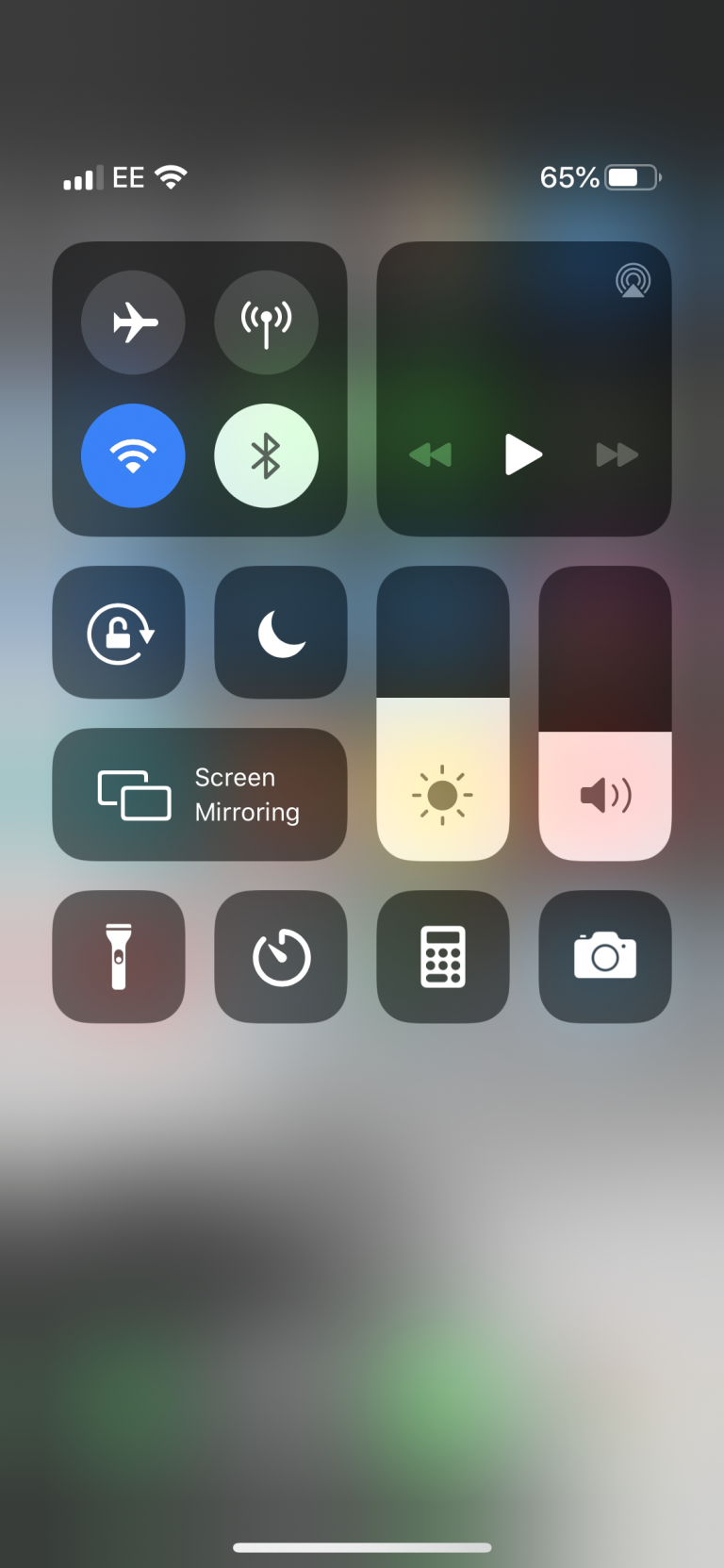This image captures a detailed screenshot of a smartphone’s control center, distinct from the home screen. The background features a sleek, reflective gray surface, adding a modern aesthetic to the interface. Multiple healthily spaced boxes reside within this control center, each containing specific icons that allow for quick access and control of various functions.

On the left, a small box contains an icon depicting an airplane, indicating the airplane mode toggle. Adjacent to this are two more icons—one likely Wi-Fi-related and below them, a recognizable blue circle for Wi-Fi, and another circle for Bluetooth. These icons are all housed within a single box, suggesting they are grouped together for convenience.

Another box displays a music control panel, complete with arrows representing rewind and forward options, as well as a play button, allowing users to manage their media playback effortlessly. There's also a box with a lock icon, hinting at an option to lock the screen or device.

Further boxes include controls for night mode, screen mirroring, brightness adjustment, and audio volume. Below these, individual boxes offer functionalities for the flashlight, power, calculator, and camera features.

At the top of the screen, standard status icons are visible, showing the battery level at 65%, Wi-Fi signal strength, and other essential notifications.